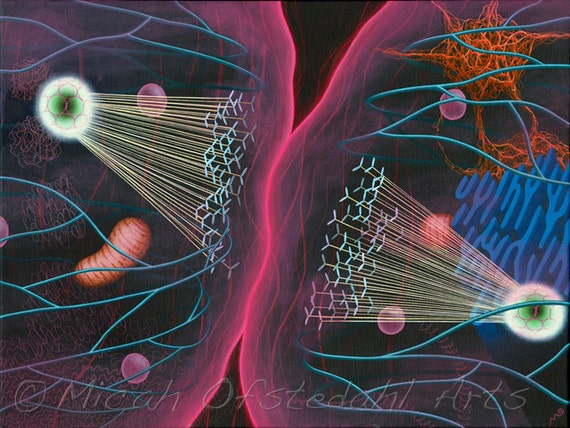The image depicts an artistic rendering that resembles microscopic organisms. Two large, interconnected circles dominate the composition, appearing as fluid cells merging together. The left cell features a central white sphere with a green core and radiating tendrils, amidst floating blue tendrils and various oblong and spherical shapes. Similarly, the right cell also contains a central white sphere with a green core and tendrils, though it is distinguished by an additional maze-like blue structure and an orange, string-like mass above it. The image is awash with a vibrant palette, including purplish pink, light blue, red, pink, green, black, and orangish red. Intricate details like blue wire-like circles, pink bubbles, and small worm-like figures add complexity to the scene. Text at the bottom credits the artwork to Micah Ostendale, Ostendale Arts.